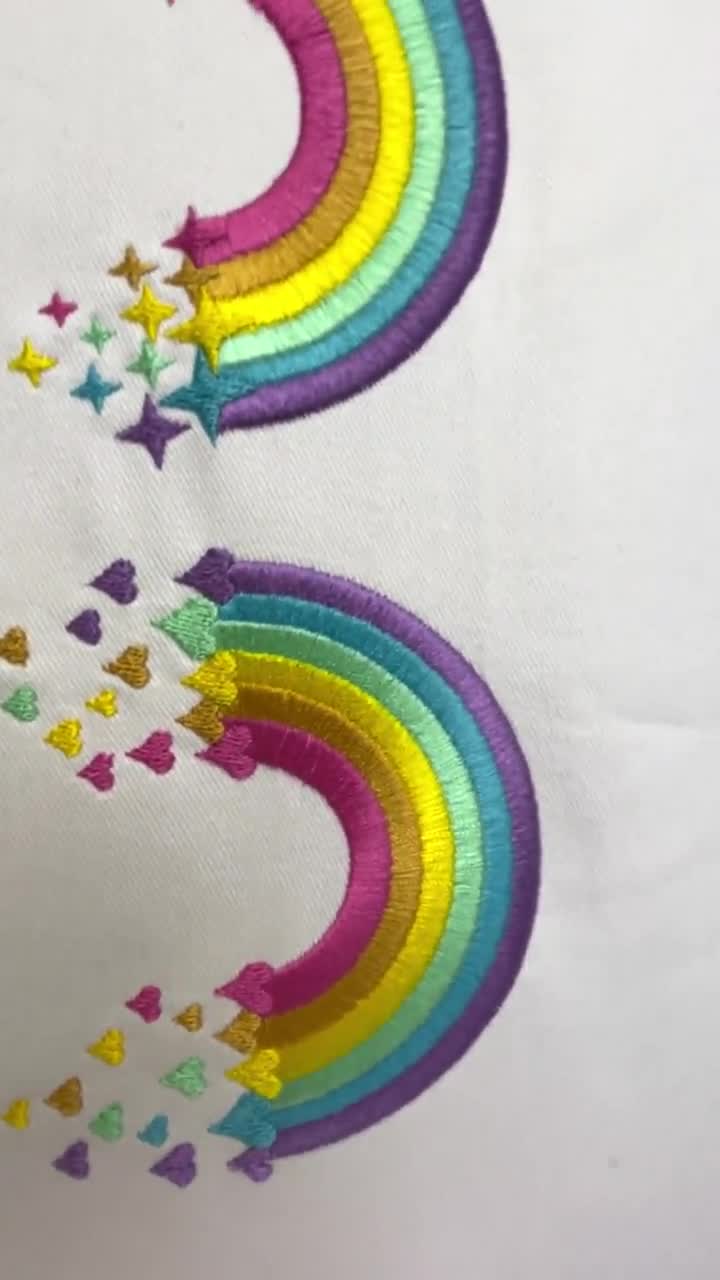This portrait-oriented color photograph captures two vertically aligned, embroidered rainbows on a white linen background. The rainbows are turned on their sides, with the arcs facing the right and the flat bases towards the left. Each rainbow showcases a vibrant spectrum of colors, from red, orange, yellow, green, blue, to violet. The top rainbow is adorned with four-pointed star embroidery at the ends of each colored section, and beneath these stars are smaller stars arranged in a triangular pattern. The bottom rainbow features heart-shaped embroidery, with each colored section ending in a cascade of smaller hearts. Both rainbows are set closely together with a small gap of space in between, highlighting the intricate details and ornate stitch work. The delicate designs and vibrant hues against the stark white background give the piece a sturdy yet aesthetically pleasing appearance, emphasizing the artistic craftsmanship of the embroidered quilt.